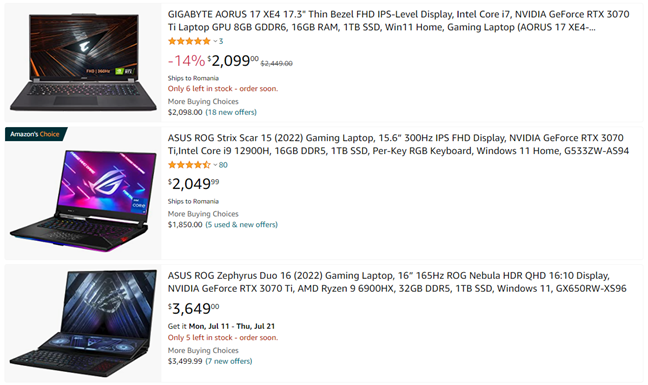The image displays three stacked laptop computers, each with detailed descriptions of their specifications and prices:

1. **Top Laptop**: 
   - **Model**: Gigabyte AORUS 17 XE4
   - **Screen**: 17.3" thin-bezel FHD IPS-level display
   - **Processor**: Intel Core i7
   - **Graphics**: NVIDIA GeForce RTX 3070 Ti laptop GPU
   - **Memory**: 16GB GDDR6
   - **Storage**: 1TB SSD
   - **Operating System**: Windows 11 Home
   - **Usage**: Gaming laptop
   - **Price**: $2,099 (14% discount)
   - **Shipping**: Available to Romania only
   - **Stock**: Only six units left, urging quick purchase
   - **Alternative Price**: $2,998
 
2. **Middle Laptop**:
   - **Model**: ASUS ROG Strix Scar 15 (2022)
   - **Screen**: 15.6" 300Hz FHD IPS display
   - **Graphics**: NVIDIA
   (Further details cut off in the provided content)

3. **Bottom Laptop**:
   - Not enough information is provided to describe the third laptop.

The image emphasizes urgency in purchasing the top laptop due to limited stock and availability to specific locations, with competitive buying choices provided.